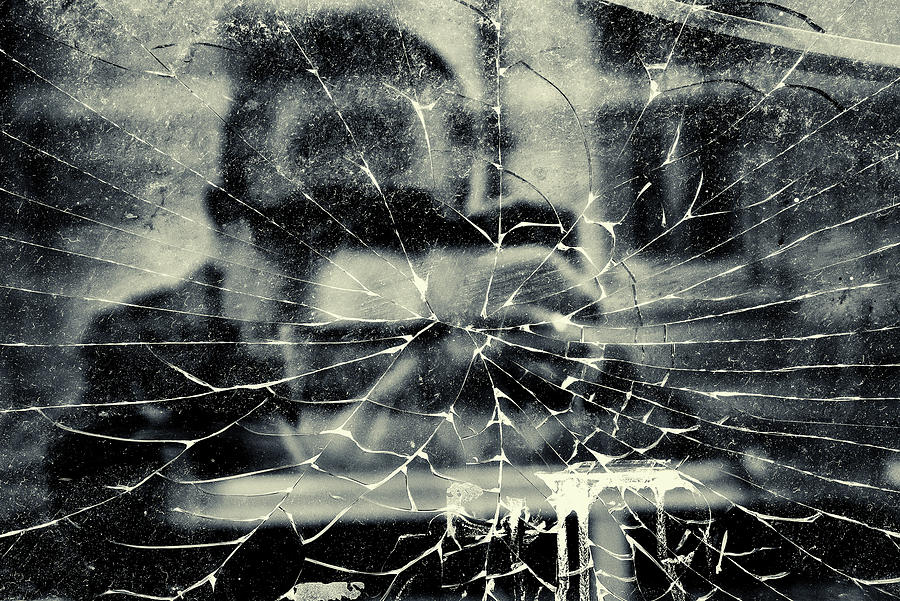This black and white photograph captures an intricate, spiderweb-like crack on a windowpane, spanning the entirety of the image. The shattered glass originates from a central point and extends outward like a web, with the white crack lines creating an intricate pattern across the surface. Through the cracked glass, the blurred reflection of a man wearing sunglasses and a black coat can be seen, holding an older rectangular digital camera pointed at the viewer. The man has very short hair and is partially obscured by the complexities of the glass. Ambient reflections behind him suggest the setting may be adjacent to other storefronts or buildings. Additionally, there is a blurred table, possibly chrome-colored, along with indistinct shapes indicating the window's frame. A black horizontal line and the break in the window where it could be pushed open are also visible, adding further depth to this multifaceted image.